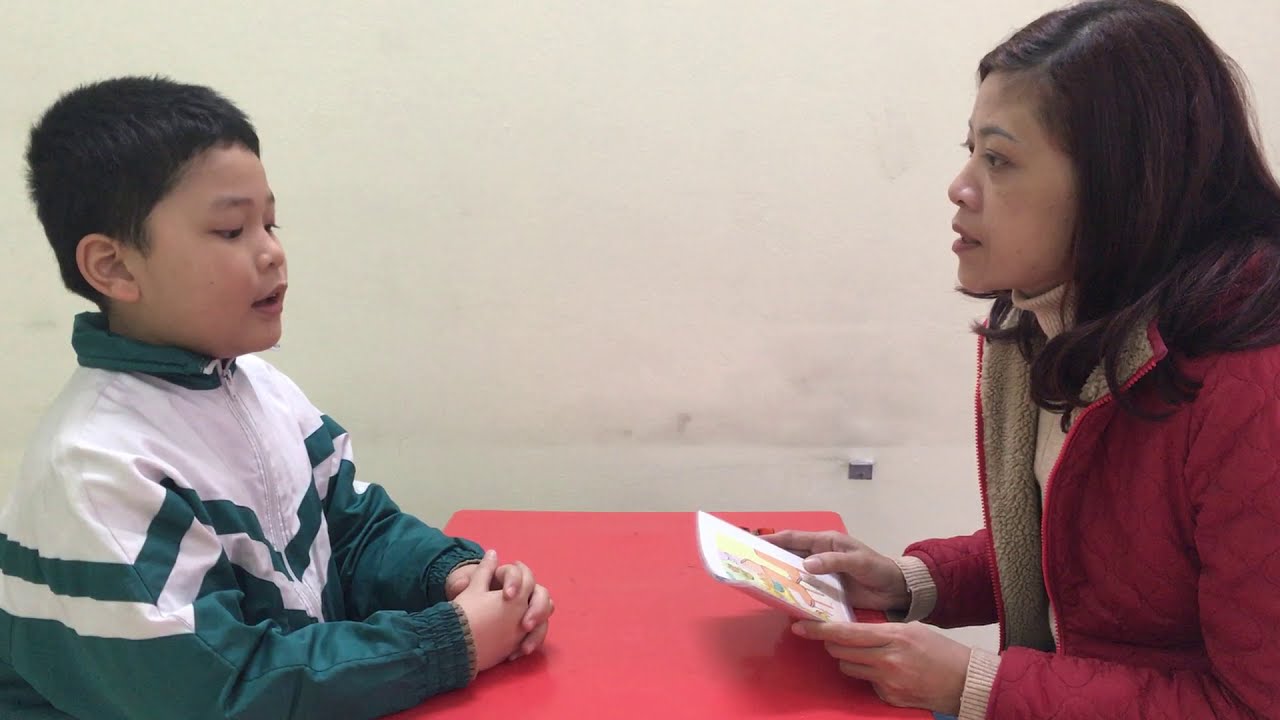In this indoor photograph, a scene unfolds between two individuals of Asian descent, set against a white background wall, likely made of some sturdy material like cement or brick. On the right side of a small, child-sized red table, sits an adult woman with long dark hair. She is dressed in a red jacket over a white shirt, and possibly wears a green scarf. Her attire suggests she could be a teacher or a therapist, engaged in an educational or therapeutic session. She is holding a white card, adorned with orange, yellow, and blue markings, and appears focused on the young boy seated opposite her.

The boy, positioned on the left side of the table, has dark hair and fair skin. He is dressed in a green and white windbreaker, with green sleeves, a white upper part featuring a green zigzag band, and a green collar. His hands rest purposefully on the table as he seems to be responding to a question from the woman. There is an air of interaction, perhaps a learning or testing scenario, as they converse. In the background, a silver electrical outlet is visible on the wall near the woman, adding subtle context to the indoor setting.